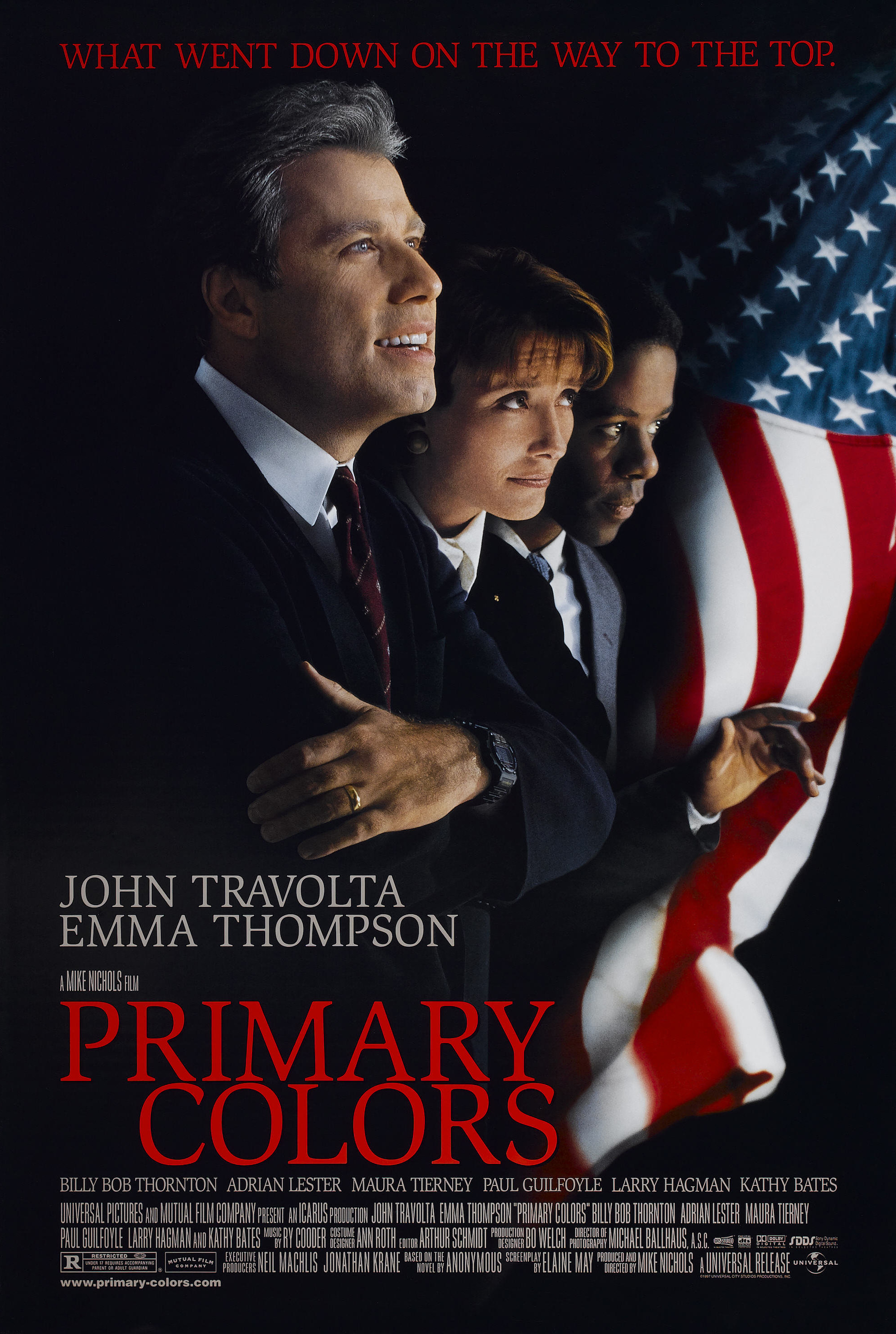The image is a movie poster with a black background prominently displaying the tagline "What went down on the way to the top" in red serif text at the top. Below the tagline is a centered photograph of John Travolta, Emma Thompson, and another person, all dressed in blue suits, looking toward the right side of the frame. John Travolta stands out with his left arm folded across his chest, wearing a wedding ring, a watch, and a red tie. An American flag with red and white stripes and a blue section with white stars decorates the right side of the poster, extending almost from the top to the bottom. The names "John Travolta" and "Emma Thompson" are displayed in white text, followed by the movie's title, "Primary Colors," which is prominently written in larger red text. Additional credits below list other stars, including Billy Bob Thornton, Adrian Lester, Kathy Bates, Maura Tierney, Paul Guilfoyle, and Larry Hagman, as well as the director, Mike Nichols. The film is noted as being rated R.